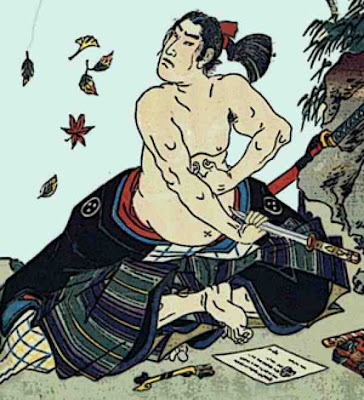This detailed illustration depicts a Japanese samurai warrior seated cross-legged in a lotus position on a sandy ground. The shirtless figure wears his garments around his waist like a skirt, exposing his stern, focused expression. He has black hair tied back with a red ribbon into a ponytail. His right hand grasps a short sword, poised towards his abdomen, suggesting an imminent ritual suicide. A white piece of paper with writing lies in front of him on the ground, accompanied by a narrow yellow object. The background is rich with detail: leaves in red, yellow, and green hues float through the air against the light blue sky. To the right, tree branches extend over a rocky cliff, and to the upper left, there is an expanse of blue sky. The left side also shows a mountain, enhancing the scene's outdoor, rugged terrain. Additionally, a longer sword in a red sheath is visible near the tree branches, adding to the warrior's solemn presence in this animated scene.